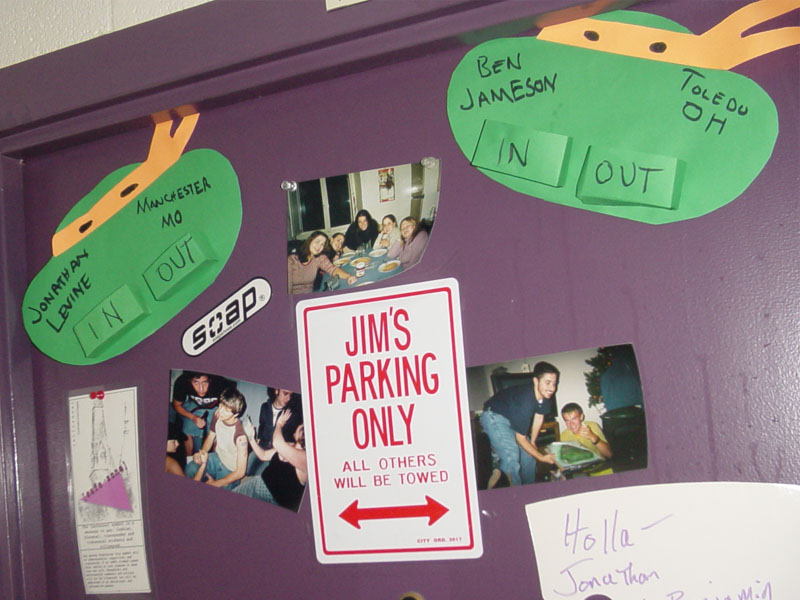The photograph shows a purple-painted, wood-like bulletin board resembling a dorm room door. The top corners of the board feature handmade construction paper crafts resembling Teenage Mutant Ninja Turtle heads. On the left side, the paper craft is labeled "Jonathan Levine, Manchester, MO, In-Out," and the right side reads "Ben Jameson, Toledo, Ohio, In-Out." Centered on the board is a humorous parking sign stating "Jim's parking only, all others will be towed." Below this sign are three photos of college students: the top one shows them gathered around a table with food, the left depicts them enjoying a party, and the right captures someone serving food, possibly pizza. Additionally, there's a handwritten note in the bottom right corner that reads, "Holla Jonathan."